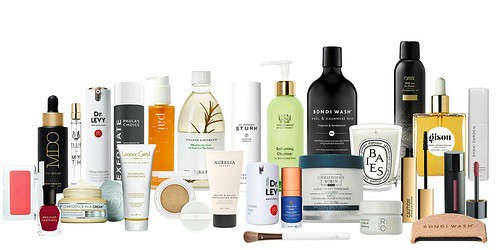The image showcases an extensive collection of approximately 20 cosmetic and skincare products arranged on a surface. The items include a diverse range of products such as blush, mascara, moisturizer, and possibly shampoo, housed in various types of packaging such as tubes and bottles. The arrangement features two somewhat uneven rows, with the shorter items positioned in the front and the taller ones in the back. The majority of the packaging is in classic black and white tones, though these colors are interspersed throughout the image, creating a visually balanced composition. Notably, nearly all the items are encased in plastic. Some products, like the blush and foundation, have transparent lids allowing the product inside to be visible, while most others remain opaque. One of the bottles is transparent enough to see its contents, adding a layer of visual interest to the assortment.